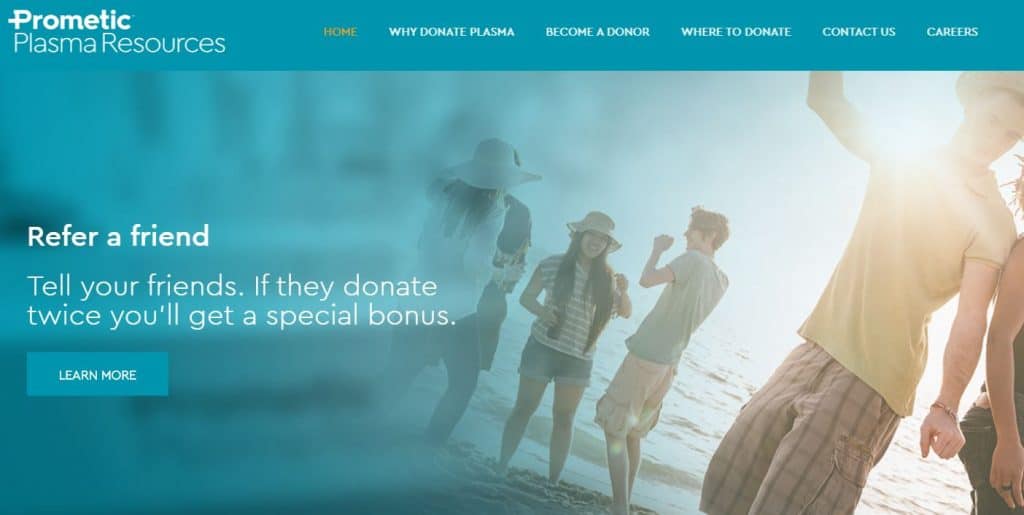The screen capture of the ProMedic - Plasma Resources website shows a well-organized homepage designed to encourage plasma donations. In the upper left corner, the website's name, "ProMedic," is prominently displayed with its tagline "Plasma Resources" below it. 

The top navigation ribbon features key sections: "Why Donate Plasma," "Become a Donor," "Where to Donate," "Contact Us," and "Careers," providing users with easy access to important information.

The main background image features a group of young people on a beach, seemingly enjoying a sunrise. The scene likely depicts individuals in their late teens to early 20s, capturing a moment of leisure and camaraderie. The right side of the image shows these friends backlit by the rising sun, creating a warm, inviting atmosphere despite making their faces somewhat difficult to see.

An overlay on the left side of the image prominently displays the text "Refer a Friend." Below this, it reads, "Tell your friends: If they donate twice, you'll get a special bonus." A "Learn More" button is located beneath this message, encouraging users to find out additional details about the referral program.

The use of a professionally taken photograph, with strategic blurring on the left to highlight the overlay text, effectively draws attention to the referral incentive, while the inviting image of young people enjoying a beach setting adds a relatable and aspirational touch to the overall website design.